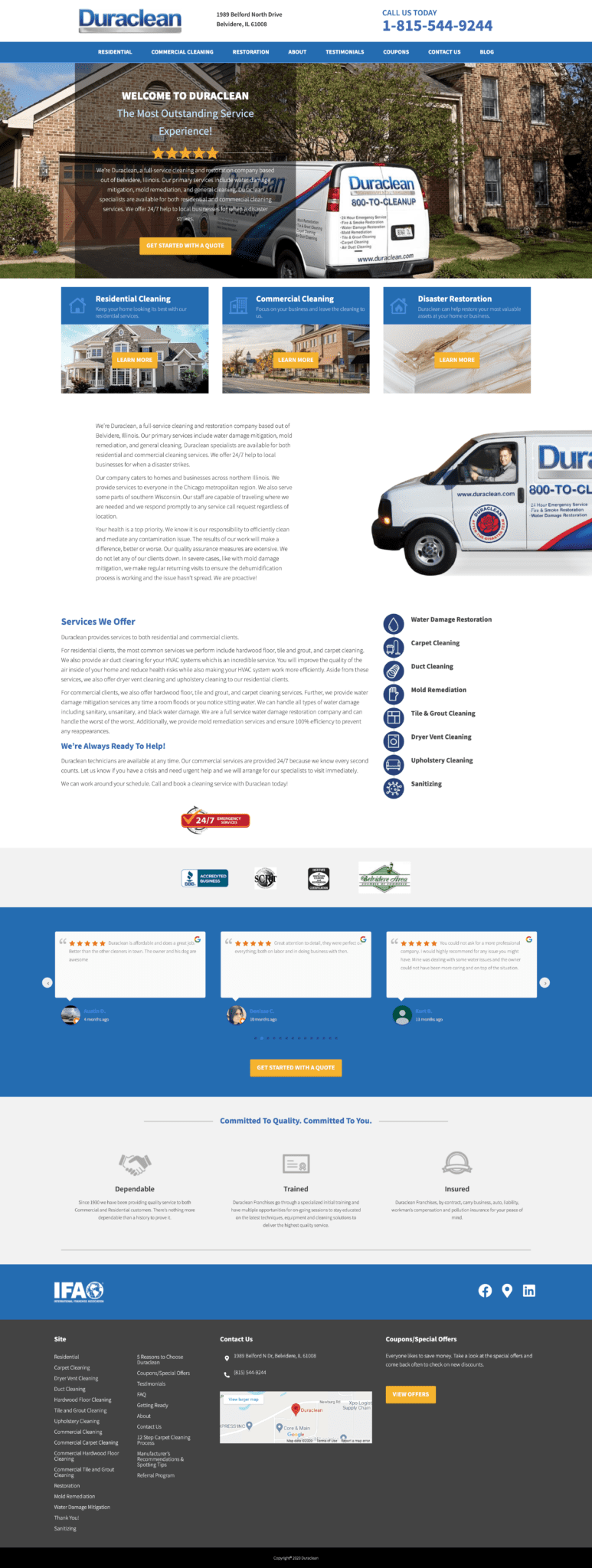The image is a screenshot of a smartphone displaying the Duraclean website. At the top, the site prominently features the Duraclean logo and a contact phone number for services within the United States. Below the header, a menu banner provides clickable options for various sections of the site. The background of the banner displays a Duraclean van parked in the driveway of a residential home near the garage, conveying the company's reliability and on-site service.

Superimposed on this background is a pop-up that reads, "Welcome to Duraclean. The most outstanding service. Five-star rated." This message highlights the company's commitment to excellence and customer satisfaction. Beneath the pop-up, there's a paragraph of text that is too small to read, followed by a gold banner with white lettering, possibly leading to more information or customer testimonials.

The main section of the website features three clickable options: "Residential Cleaning," "Commercial Cleaning," and "Disaster Restoration," the latter covering services for fire, flood, and other emergencies. Additional imagery includes another view of the Duraclean van, showcasing the company's branding and professionalism. Various banners on the site tout their high service standards and display customer testimonials. A feature to locate the nearest Duraclean service and schedule an appointment is also available, emphasizing convenience and accessibility for prospective clients.